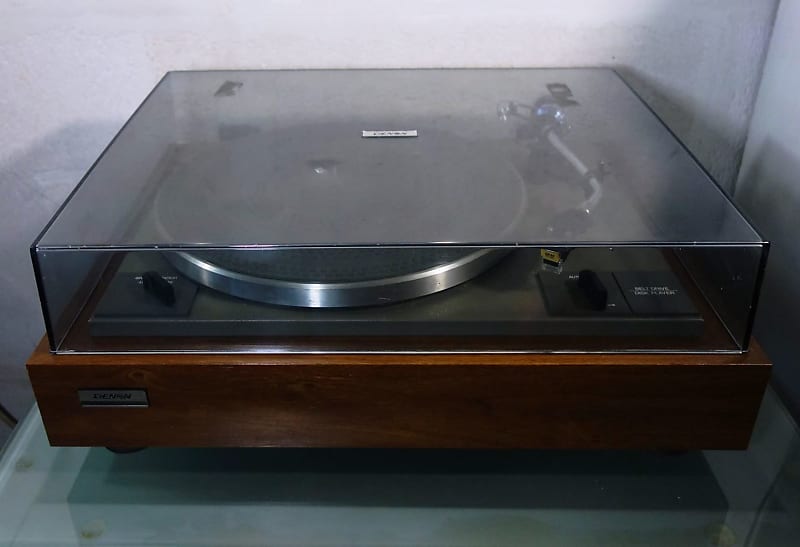This image showcases a vintage record player, likely from the 1970s, with a well-crafted wooden frame stained in a rich mahogany color. It features a square base with short legs. Its lid is made of smoked, tinted plastic, matching the dimensions of the base and can either be lifted up to lean backward or fully removed via hooks at the back. The central turntable, where vinyl records are placed, consists of a circular disc with a black rubber top and chrome metal sides. Controls include two knobs on the front for adjusting the speed between 33 and 45 RPM. Positioned on the right side is a curved metal arm ending in a black-tipped needle, which automatically lifts, plays the record, and returns to its resting position when activated. A small silver plaque, though unreadable in the image, is located at the bottom left corner of the wooden frame, indicating the brand. The record player is set against a white wall on a light, bluish-green surface.